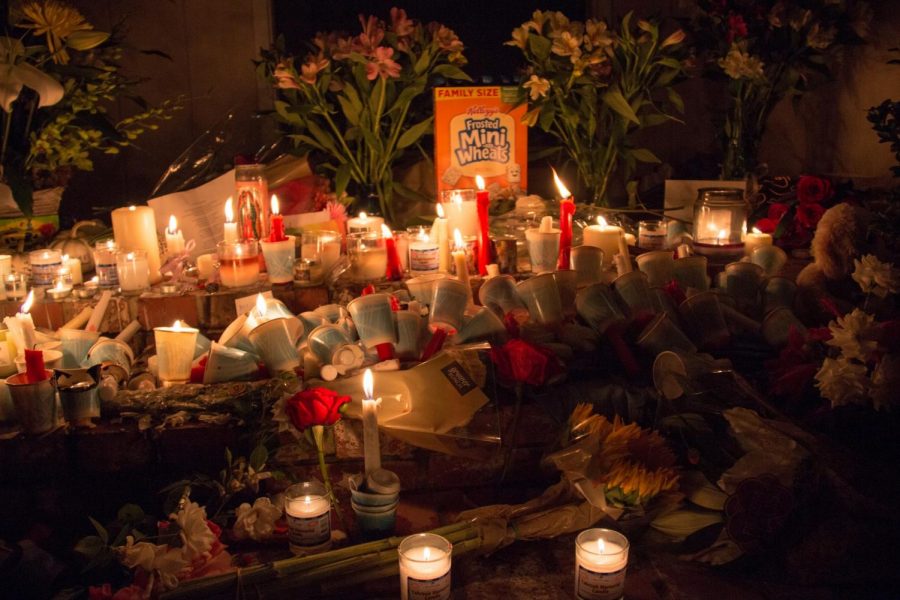This is a color photograph taken at night, depicting an outdoor vigil or memorial. The central focus of the image is a box of Kellogg's Frosted Mini-Wheats placed at the top middle, marked with the text "family size". Surrounding the cereal box are multiple white and red candles, some of which are lit, creating a somber and reflective ambiance. There are also bouquets of flowers in colors such as pink and white arranged around the scene. Additional details include scattered books and papers, enhancing the sense of a personal memorial. The colors in the image range from orange, green, yellow, and white to brown and red, contributing to the overall solemn yet heartfelt atmosphere.